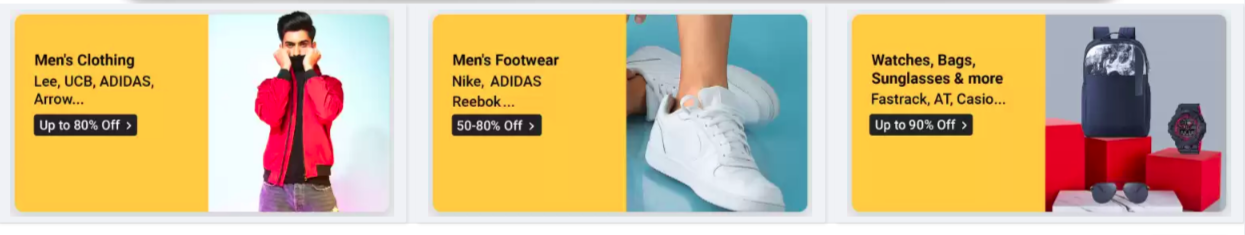This screenshot primarily features a white background with a thin gray line running horizontally across the top. Below this line are three rectangular images arranged in a row, showcasing various promotional offers.

1. **First Image (Left)**: The leftmost image is rectangular and horizontally extended. The left half of this image is a bright yellow box containing black text that reads "Men's Clothing: Lee, UCB, Adidas, Arrow." Additionally, there is a small black box with white text stating "Up to 80% Off." The right half of the image features a young man with black hair, wearing a white and red jacket over a black turtleneck, paired with jeans.
 
2. **Second Image (Center)**: The center image also has a yellow box on its left half, which reads "Men's Footwear: Nike, Adidas, Reebok." It also contains a black box with white text indicating "50-80% Off." This section draws attention to discounted footwear from popular brands.
 
3. **Third Image (Right)**: The rightmost image highlights various accessories with the text "Watches, Bags, Sunglasses and More: Fastrack, AT, Casio." It includes a small black box with white text that advertises "Up to 90% Off." This section is dedicated to significant discounts on different accessories from well-known brands.